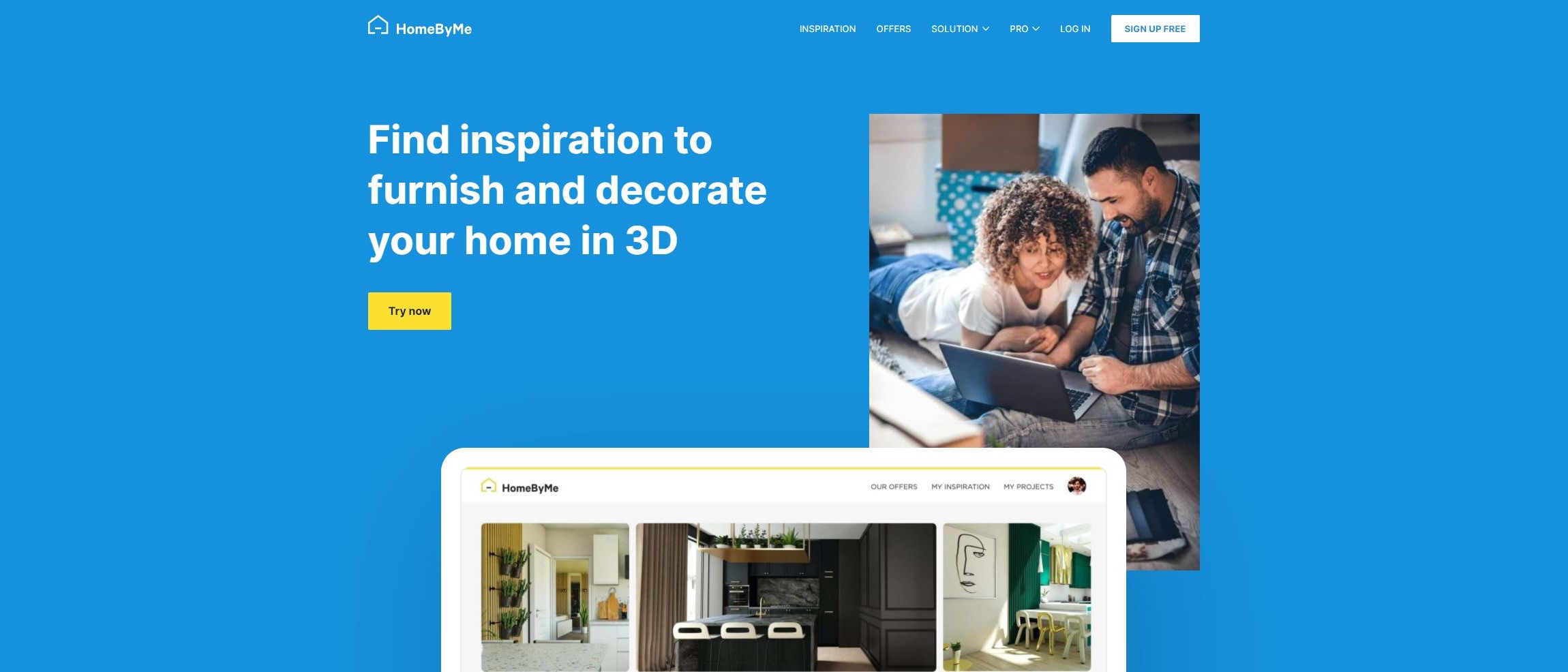The image displays a vibrant website interface for "Home by Me," featuring blue text with the brand name. The page offers solutions for creating 3D home decor and furnishing inspirations, with a prominent call-to-action button in a white rectangle labeled 'Sign Up Free.' Above it, another message in white text reads 'Find inspiration to furnish and decorate your home in 3D.' A bold yellow rectangle invites users to 'Try Now.'

On the right side of the interface, an illustration of a person with curly hair wearing a shirt appears prominently. Below this figure, there is a depiction of a laptop, reinforcing the digital and interactive nature of the platform. 

The interface is organized with yellow-line dividers categorizing sections like 'Our Offers,' 'My Inspiration,' and 'My Projects,' ensuring easy navigation. 

The background imagery is a beautifully staged room with large green leaves on the walls, potted plants, and a white door. There is a table dressed with decor elements and a brown curtain adding warmth to the setting. Above, pots and green plants are arranged decoratively.

Walls are painted brown, complementing the central island table which is surrounded by chairs, creating a cozy yet modern dining area. To the right, a painting adorns the wall, adding an artistic touch. The overall aesthetic is modern-chic with a blend of nature-inspired elements, making this interface inviting and inspirational for users looking to decorate their homes.